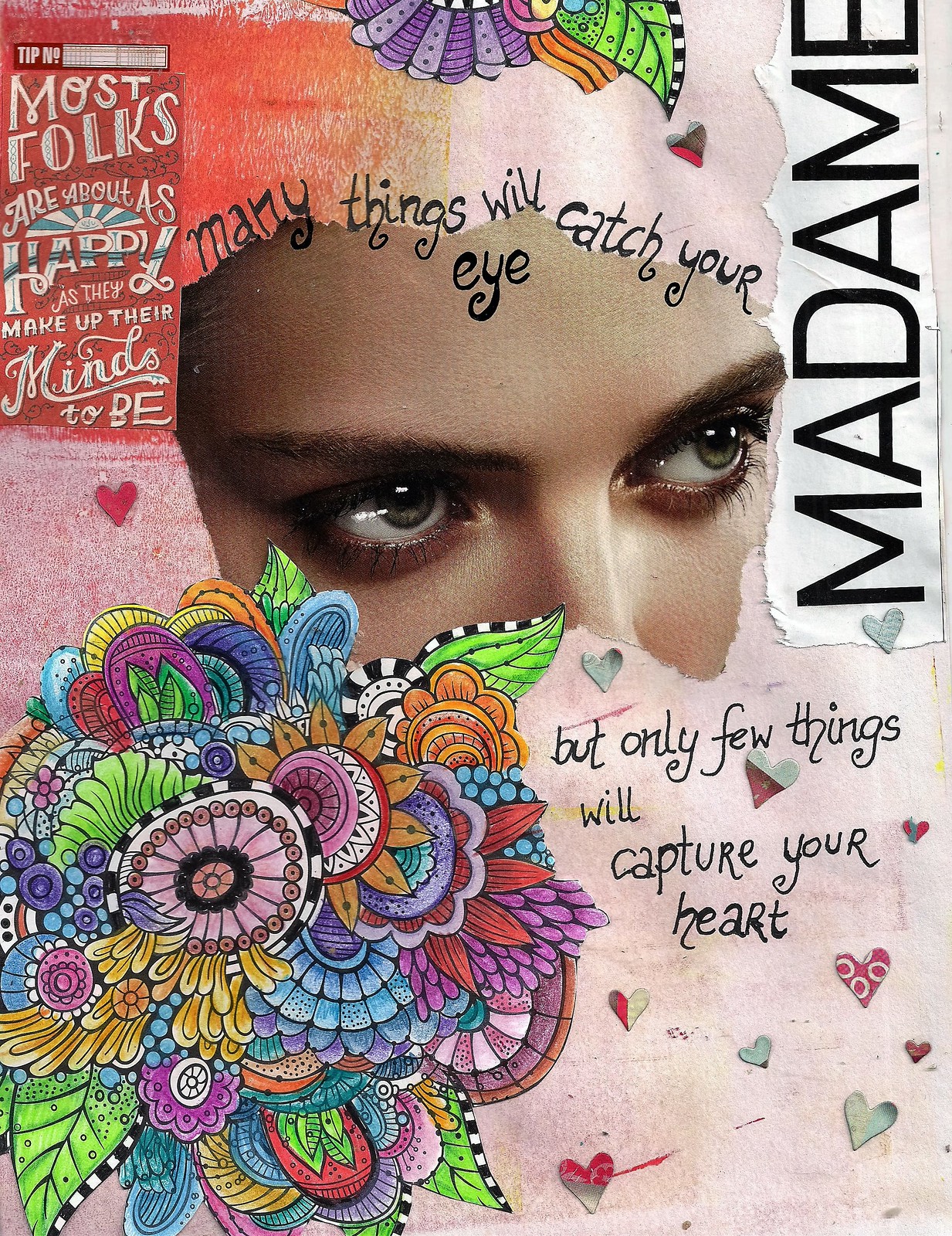The image appears to be an abstract, rectangular artwork or possibly a montage influenced by a 1960s psychedelic style. At the center of the image, there's a rough-edged cut-out of the top half of a woman's face, showcasing her light green eyes and forehead up to just above her nose bridge. The woman, who has a lighter complexion and is gazing to her left, has her hairline cut off. Handwritten black text above her forehead reads, "Many things will catch your eye," while below her face it continues, "but only a few things will capture your heart." 

On the right side, the word "MADAME" is written vertically in all capital letters, accompanied by a silver heart at its base. A smaller cut-out text box on the left contains an inspirational quote: "Most folks are about as happy as they make up their minds to be." The artwork features numerous vibrant elements, including various colored hearts scattered around and a hand-drawn bouquet of flowers, colored with what appears to be colored pencils, in the bottom left corner. Additional drawings of psychedelic flowers extend from the center towards the bottom, enhancing the whimsical and eclectic nature of the image.